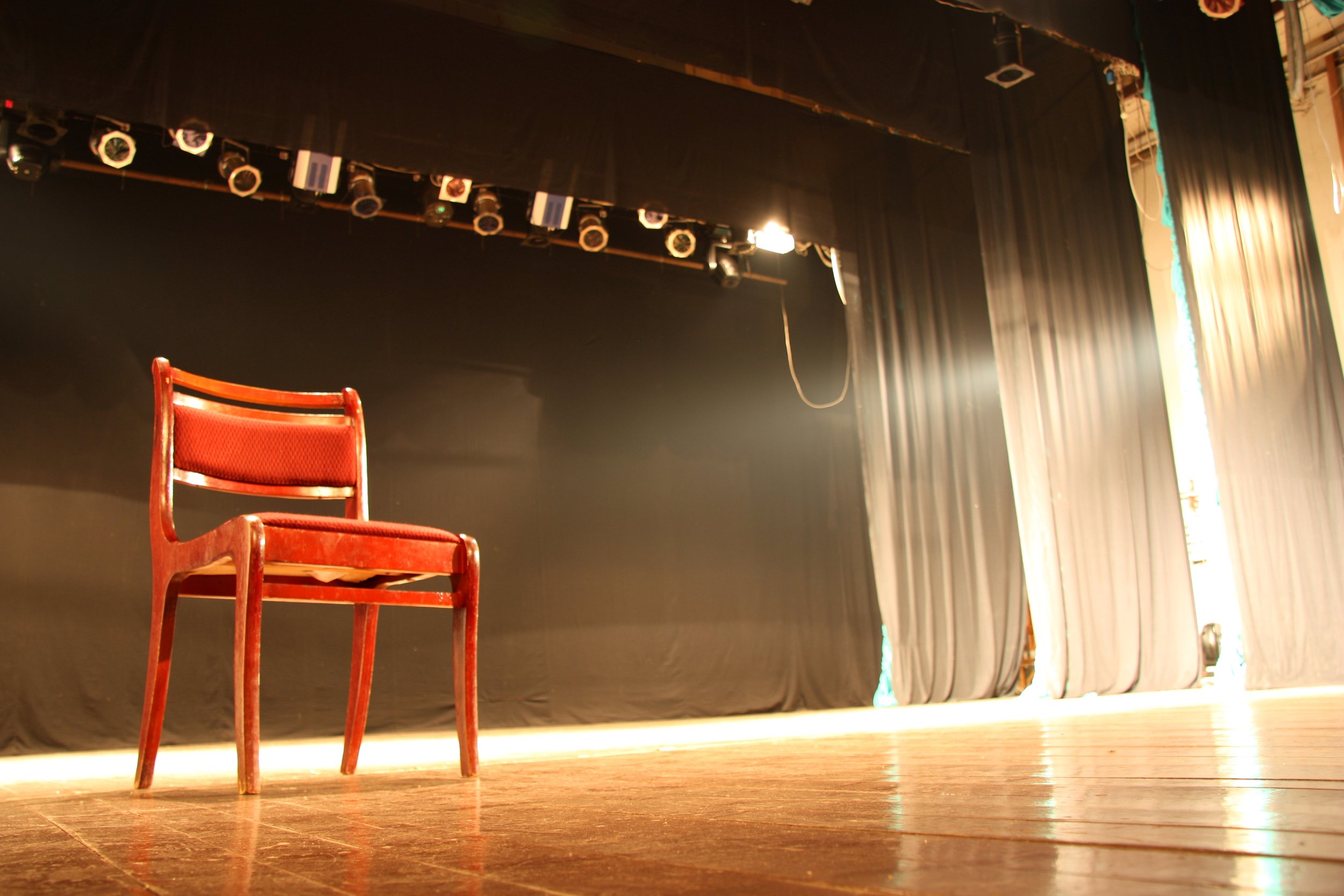This detailed color photograph showcases a polished, varnished wooden stage, glistening under multiple light sources. Dominating the scene is a solitary red wooden chair stationed to the left, facing the viewer. The stage's shininess is accentuated by a combination of dim and active lighting, including a prominently lit stage light from above and an illuminated beam from the left side. On the right, the stage is framed by four levels of curtains—three of these black or beige curtains drawn back to reveal a backdrop. The ceiling features an array of stage lights, most dimmed except one, casting a gentle glow across the floor. This image captures a silent, yet evocative moment, emphasizing the stark loneliness of the red chair amidst the expansive, empty theatrical stage.